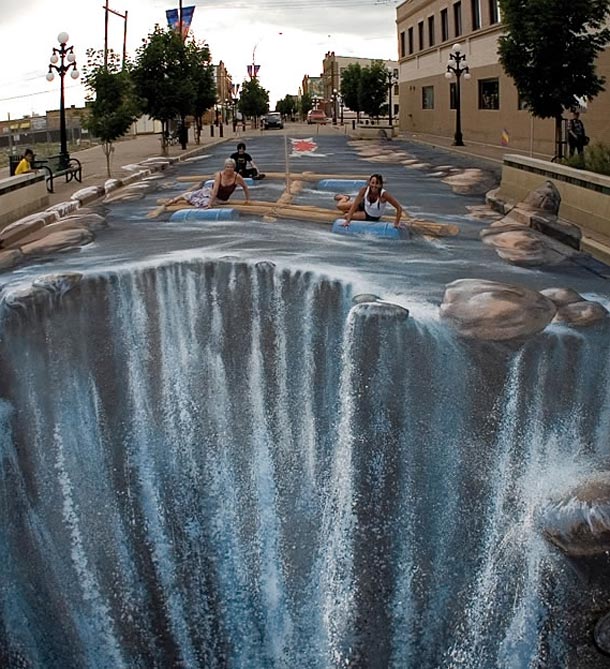A vividly detailed, vertical image portrays a surreal scene of a city street transformed into a cascading waterfall. The central focus is on three individuals – a dark-haired woman, a light-haired woman, and a man – smiling as they sit on a simplistic rescue raft adorned with a white flag and flotation devices, seemingly floating on blue water. This imaginative artwork uses a chalk painting technique to create the lifelike illusion of a street turning into a river, complete with large painted boulders and unnatural shadows. Alongside the street, a person in a yellow shirt sits calmly on a park bench while others walk by, observing the scene. Streetlights and parked cars line the sidewalks, framing this fantastical tableau that bridges the gap between the real and impossible.